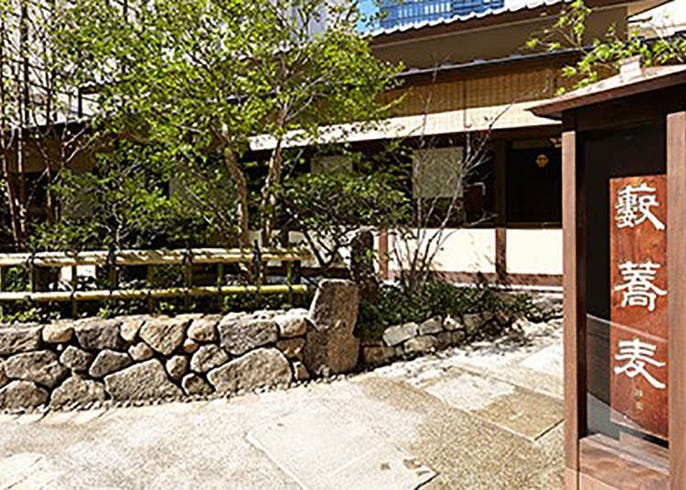The somewhat blurry photograph captures the front of a multi-layered Pagoda-style building, with distinct architectural elements receding from view. The building, appearing white and brown, has four distinct layers, with the topmost being a blue square checkered design. In the foreground is a gray concrete sidewalk leading to a short rock wall made of variously-sized, piled stones. This wall is part of an island that hosts small trees, greenery, and a fence separating it from the pathway. Prominently, to the right foreground, stands a wooden kiosk with a roof, featuring three large, vertically-arranged, pictographic Asian characters painted in white, likely Japanese or Chinese. The scene is further complemented by bushes, other plants, and a large green tree sprouting in the middle ground, adding a touch of nature to the urban setting. Above and behind the pagoda-style building, a portion of a modern high-rise constructed from steel and glass is subtly visible, along with a glimpse of the blue sky in the upper part of the image.